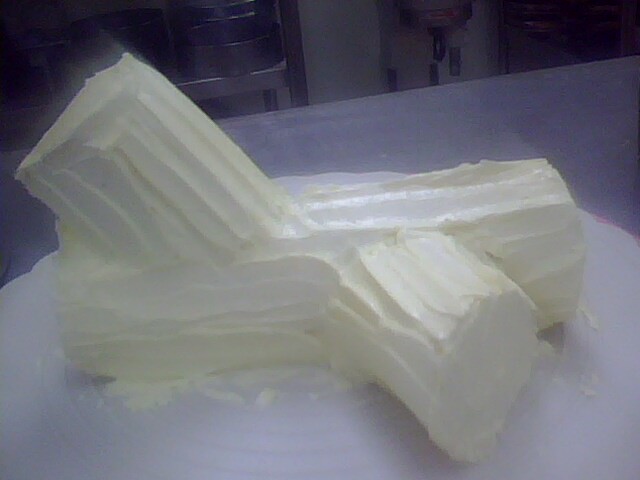The image shows a white, log-shaped object with a creamy, butter-like texture, adorned with numerous horizontal lines and grooves along its sides, suggesting it has been shaped or molded with a knife. Protruding from the main log are smaller log-shaped pieces that give the appearance of being stacked or arranged to resemble a miniature log cabin structure. The setting appears to be a kitchen, with a gray table surface below and possibly a chair in the background, hinting that this object is likely an edible item such as processed cheese, butter, or a frosting-covered dessert. The object rests on a large, white circular plate, though the overall image quality is quite blurry, especially towards the edges.